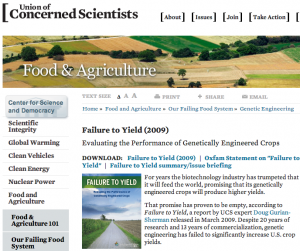**Screenshot from the Union of Concerned Scientists Website**

At the top of the screenshot, a navigation bar displays links for "About," "Issues," "Jobs," and "Take Action" on the Union of Concerned Scientists website. The header image showcases a vibrant agricultural landscape with areas distinguished by dark green, light green, and yellow hues, interspersed with trees. Below, a prominent title reads "Food and Agriculture."

On the left, a vertical menu lists various sections including: 
- Center for Science and Democracy
- Scientific Integrity
- Global Warming
- Clean Vehicles
- Clean Energy
- Nuclear Power
- Food and Agriculture
- Food and Agriculture 101
- Our Failing Food System

To the right, subcategories and resources on the topic are detailed:
- "Failure to Yield 2009"
- "Evaluating the Performance of Genetically Engineered Crops"
- Downloadable links for "Failure to Yield 2009," "Oxfam Statement on Failure to Yield," "Summary," and "Issue Briefing"

A paragraph provides context on the biotechnology industry's unfulfilled promises of higher yield genetically engineered crops. It references "Failure to Yield," a report by UCS expert Doug Kerwin-Sherman, released in March 2009, which reveals that despite two decades of research and over a decade of commercialization, genetic engineering has not significantly improved U.S. crop yields.

To the left of this write-up, an image titled "Failure to Yield" depicts a horizon with a cloudy sky. The image contrasts an area of lush, healthy crops on the left with a neighboring area of brown, deteriorating crops on the right, symbolizing the disparity in agricultural outcomes.

This detailed snapshot captures the essence of the Union of Concerned Scientists' work on evaluating the impact of genetically engineered crops on food production.